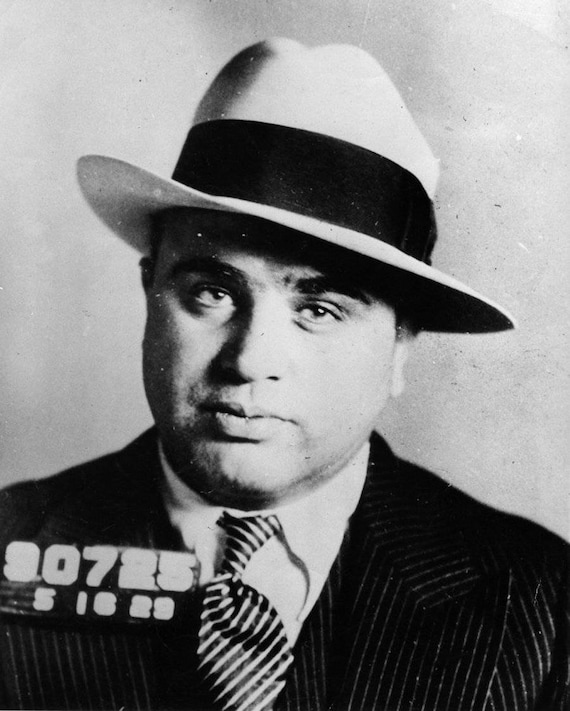This aged black-and-white photograph features a close-up mugshot of the infamous gangster Al Capone, likely taken during his incarceration in the 1920s or 30s. Al Capone stares straight ahead, wearing a distinctive white fedora with a thick black band and a slightly upturned left brim. His eyebrows are thick and bushy, and there's a visible scar near his eye. He is dressed in a dark pinstripe suit with gray stripes, a crisp white shirt, and a black and white striped tie. On the bottom left corner of the image, the prisoner identification number "90725 51629" is clearly displayed. The background is a light white wall, typical for prison mugshots. The photograph shows signs of aging, with white flecks and marks, but remains largely clear and intact.